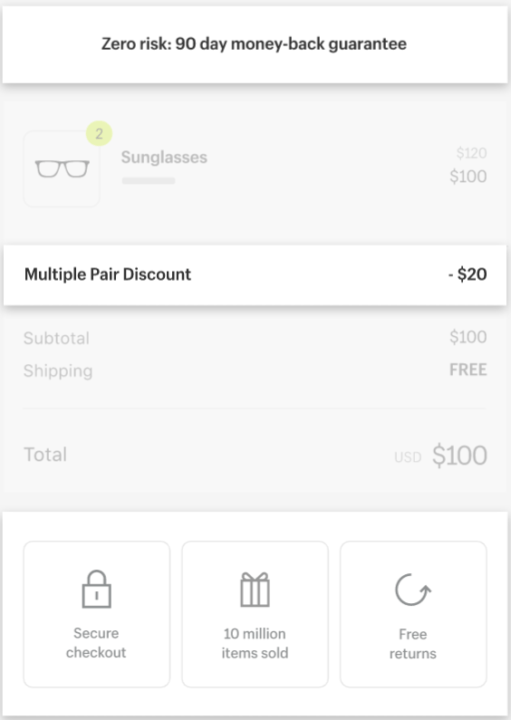**Descriptive Caption:**

The image is a detailed screenshot from an online shopping website. The overall background is a mix of white and gray tones, with important information highlighted in different sections. 

At the very top, there's a white border proclaiming a "Zero Risk, 90-Day Money-Back Guarantee." Directly below, a grayed-out background displays an image of fashionable sunglasses, accompanied by a yellow circle featuring the number "2." Adjacent to the image, the word "Sunglasses" appears, followed by a price tag of "$100" on the right.

Just beneath this section, a white pop-up rectangle indicates a "Multi-Pair Discount -20," which seems to signify a reduction in price for buying multiple items. This is followed by a gray area that’s a bit harder to discern, but it lists the "Subtotal: $100" and mentions that shipping is free. Finally, the total amount due is clearly stated as "USD $100" on the right.

At the bottom of the image, a white area features three distinct squares. The first square shows a padlock icon with the label "Secure Checkout." The second square has an icon resembling a present, with the text "10 Million Items Sold." The third square features a refresh-like icon, accompanied by the words "Free Returns."